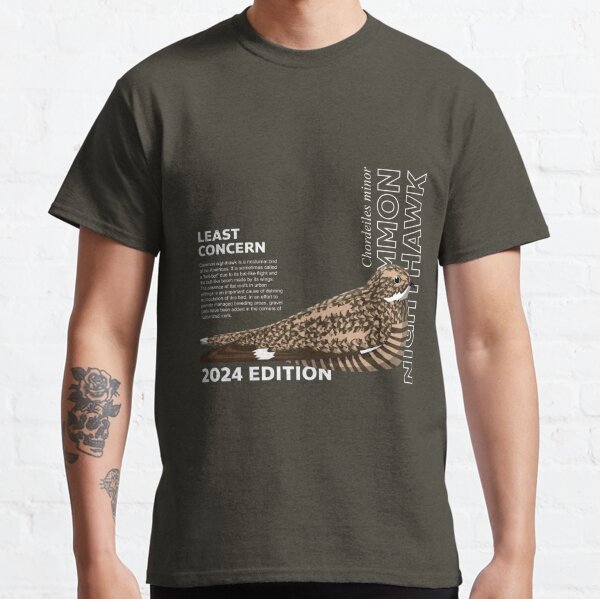The photograph features a man wearing a dark green T-shirt with a distinctive design against a white brick wall background, which fades slightly toward the upper left but maintains clear brick details toward the bottom and right side. The T-shirt features an image of a light brown bird and multiple text elements. On the left side, vertically along the chest, it reads "Least Concern" in white block letters with a paragraph of smaller, unreadable text below. Centrally, the bird is identified with the text "2024 edition" below it. Just below this text, the bird species is indicated with the scientific name "CHORDEILES minor" written sideways. The man has visible tattoos on his right forearm, including a floral design atop a skull and another tattoo partially visible, wrapping around the back of the arm. The photograph only shows his body from the neck down to the base of his hands, with a small part of his black pants visible at the bottom.